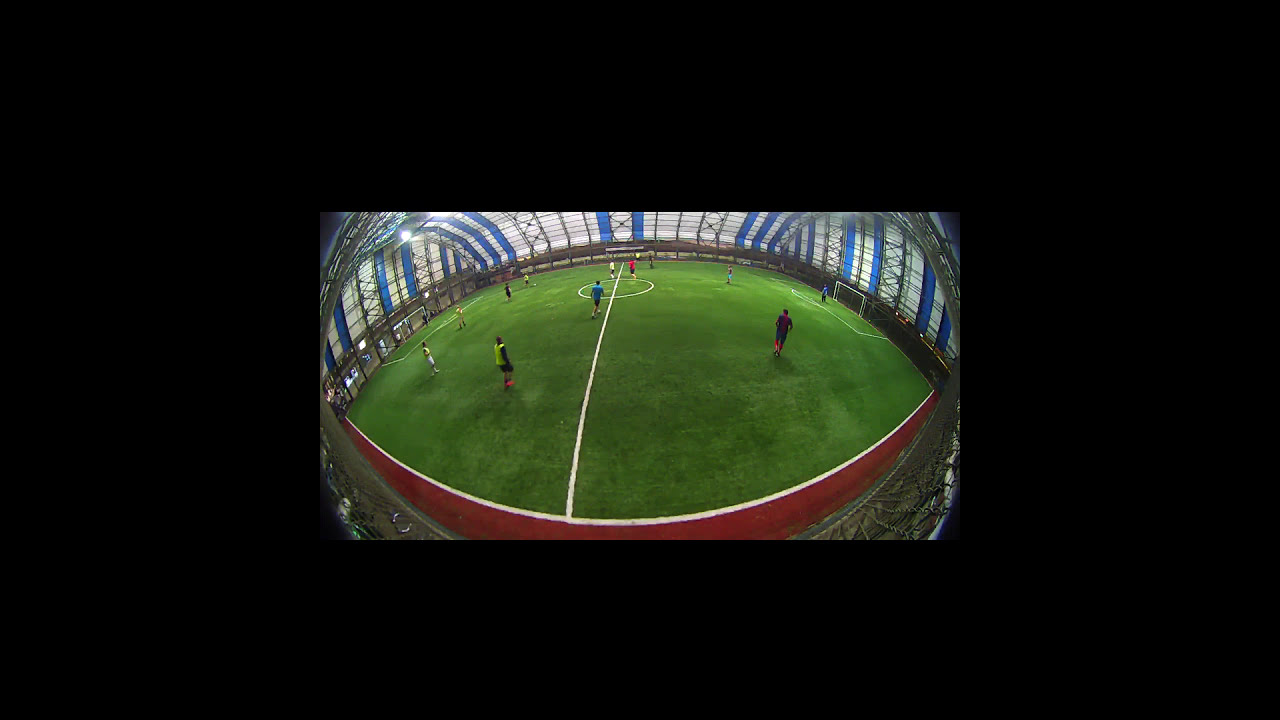The image depicts an indoor soccer field from an aerial perspective, creating a slightly oval or circular appearance, possibly due to the use of a concave or convex lens. The green field is marked with white lines, and you can see two white goals at either end. Surrounding the field is a distinct red band or track, and the structure enclosing the field features blue and white walls interspersed with black bars and silver gates. The scene is lit from above, highlighting the players scattered across the field, each wearing differently colored jerseys. The dozen or so players are engaged in a game, with one player poised to kick the ball, while others are positioned across the field. There's no visible audience, and the edges of the image fade into a black background, emphasizing the indoor setting.